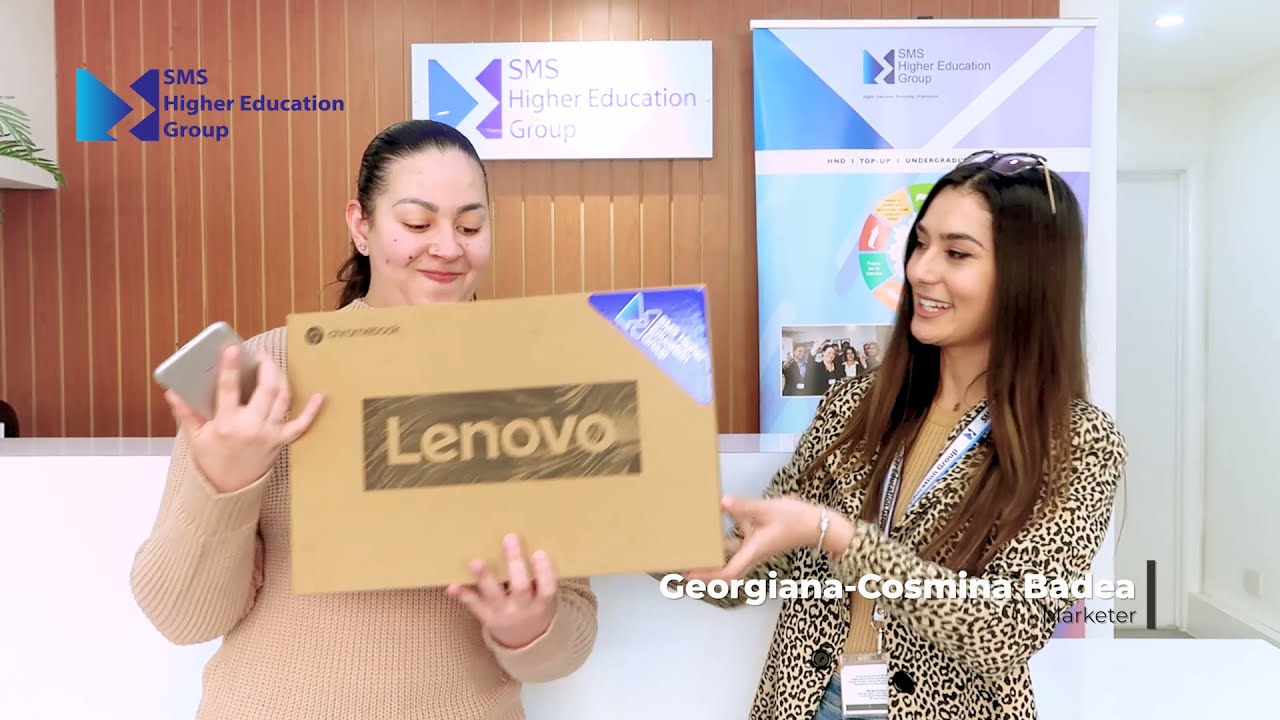The image captures a vibrant moment featuring two smiling women in a well-decorated room, likely from a TV commercial or marketing video. The woman on the left, who has white skin and black hair, is clad in a cream-colored sweater. She holds a cardboard box labeled "Lenovo" in her left hand, while her right hand grips a mobile phone, her attention fixed on the box. The woman to her right, also with white skin but sporting brown hair with sunglasses perched on her head, assists in holding the box with her left hand while her right hand supports it from behind. She is dressed in a cream-colored jacket with black patterns and has a name tag around her neck that reads "Georgiana Cosmina Badea, Marketer." Both women are beaming with joy. The background features a wall adorned with several boards, prominently displaying "SMS Higher Education Group" multiple times along with their blue logo.